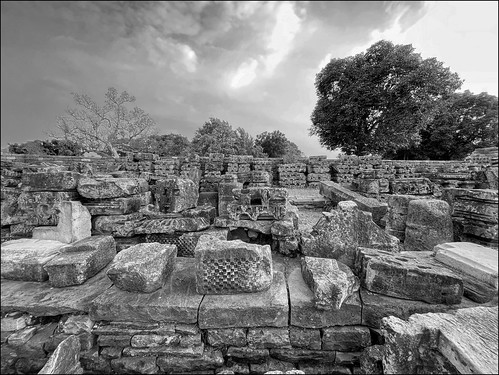This black-and-white photograph captures what initially appears to be ancient stone ruins but might also be a site where different types of stone for construction are displayed. The foreground features a detailed wall constructed of various stones, including large rectangular blocks laid horizontally, topped with an array of stones featuring diverse sizes, shapes, and textures. Some stones have patterns or divots, reminiscent of old frescoes, while others are more utilitarian, cut into lengths suitable for pathways. The background reveals a second wall built from stones with holes, giving a lighter appearance, and further back, there are signs of a courtyard or the foundation of an old building. Among the scattered stones, some are disheveled and fallen over. The setting is framed by the natural landscape, with several trees visible. To the right, there are tall trees with dark outlines, and to the left, a leafless tree stands, hinting at either old age or a winter season. The sky overhead is gray and threatening, adding to the historical and somewhat mysterious ambiance of the scene. The photograph lacks any text or human presence, focusing entirely on the interplay of stone structures and natural elements.